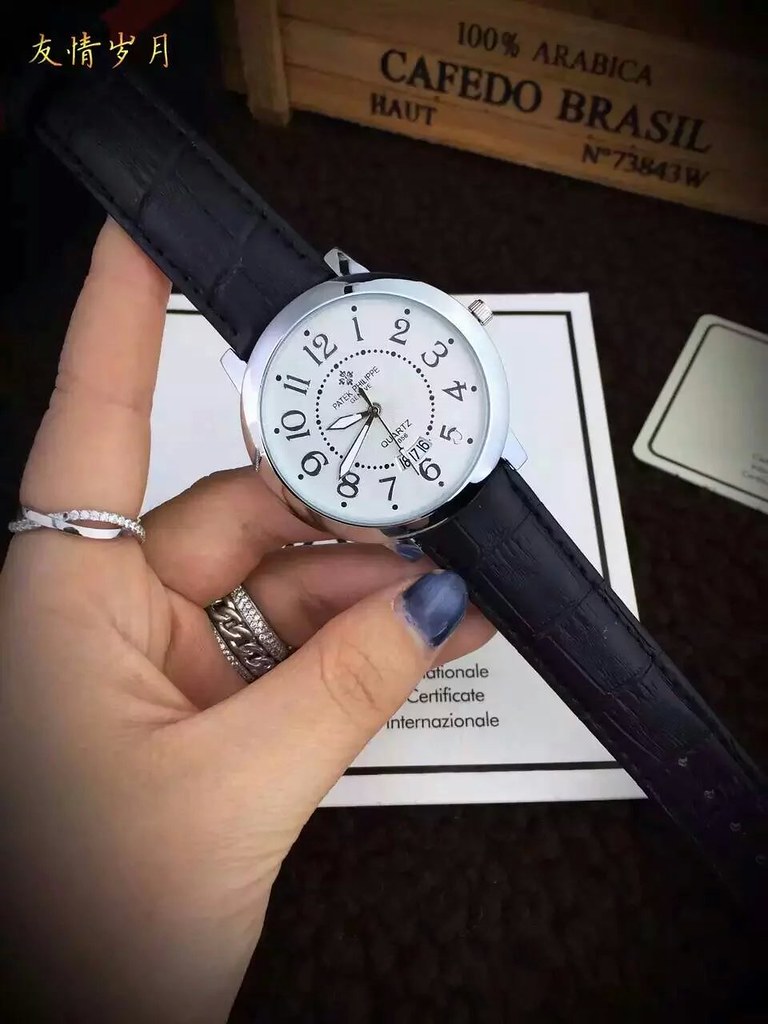This high-quality photograph features a close-up of a wristwatch held by a woman. The watch, sporting a silver bezel with a white face and black numerals, displays the current time as 9:41. It has three hands: a long white hand with a black outline, a shorter, broader hand, and a thin, long black second hand, all originating from the center. Below the "12" marker and under the hands, there is lettering that is not fully legible in the image.

The wristwatch is equipped with a dark blue leather strap that is diagonal in the composition, extending from the upper left corner off-screen and just above the right corner downward. Visible on the strap are three holes for the clasp.

The woman's hand enters the frame from the bottom left corner, with her thumb positioned along the bottom of the band. Her pinky and ring fingers support the lower part of the band, while her middle finger is under the middle part of the watch, and her index finger extends under the top part of the band. She is adorned with silver rings on her index and ring fingers, which are painted with a dark nail color.

In the background, there is a dark table surface. A white piece of paper with a black border appears near her thumb, possibly containing certification for the watch. Further back, a brown crate with black lettering reads "100% Arabica Café do Brasil." Below this in smaller lettering are "HAUT" on the left and "N73843W" on the right, with Chinese characters visible in the top left corner.